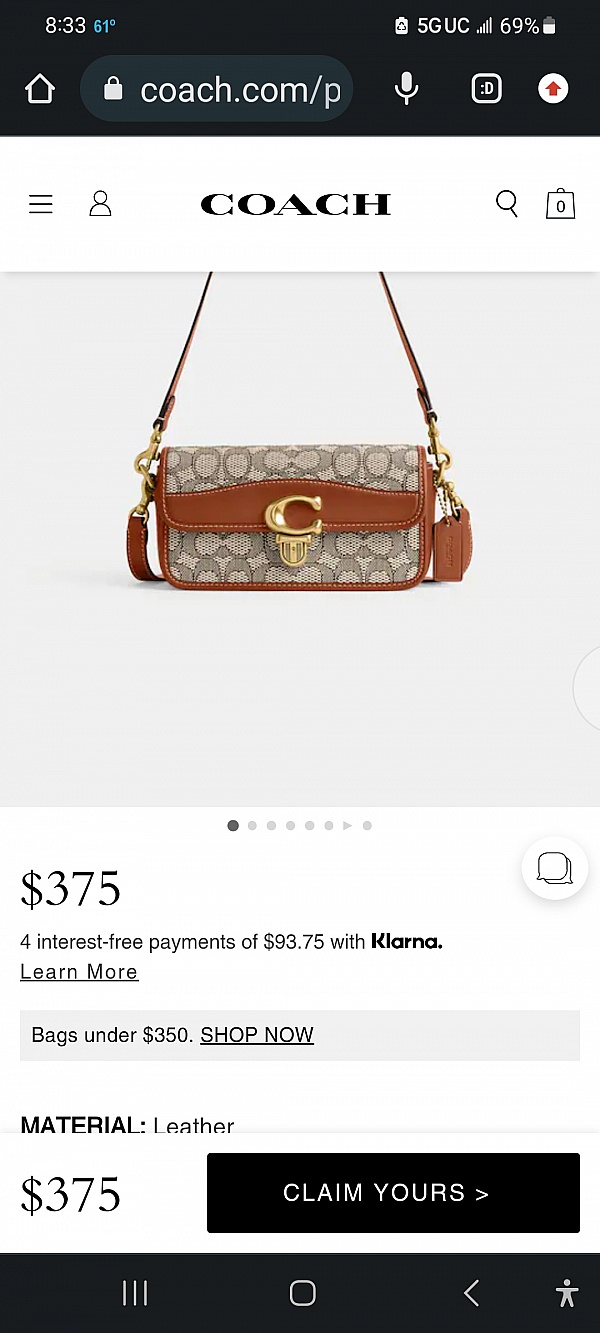Here is the cleaned-up and detailed caption for the image:

---

This screenshot showcases an online shopping interface for a Coach purse on a mobile device. At the very top is a black status bar displaying the time, temperature, battery strength, signal strength, and 5G connectivity. Immediately below, a navigation banner includes a home button, the URL "coach.com/P," and three icons: a recording icon, a “D” in the middle, and a red upward arrow.

The central portion of the screen features the brand name "Coach" prominently displayed along with a square image of the purse. There are icons on either side of the purse image for additional interaction. Multiple small dots beneath the image indicate the presence of additional screens that can be navigated through.

Following this section, the price of the purse is listed as $375 on the left side. On the right, there is a chat icon for customer support. Below the price, a message informs users that they can make four interest-free payments of $93.75 with Klarna. A clickable "Learn More" link is available for additional information.

A gray banner beneath this section advertises "Bags under $350" with an underlined "Shop Now" call to action. The materials of the purse, listed as coal and leather, are noted below, and although partially obscured, there is a transition to a white banner. This banner reiterates the $375 price on the left, with a black "Claim Yours" button on the right for immediate purchase. At the very bottom of the screen, standard Android navigation icons are visible.